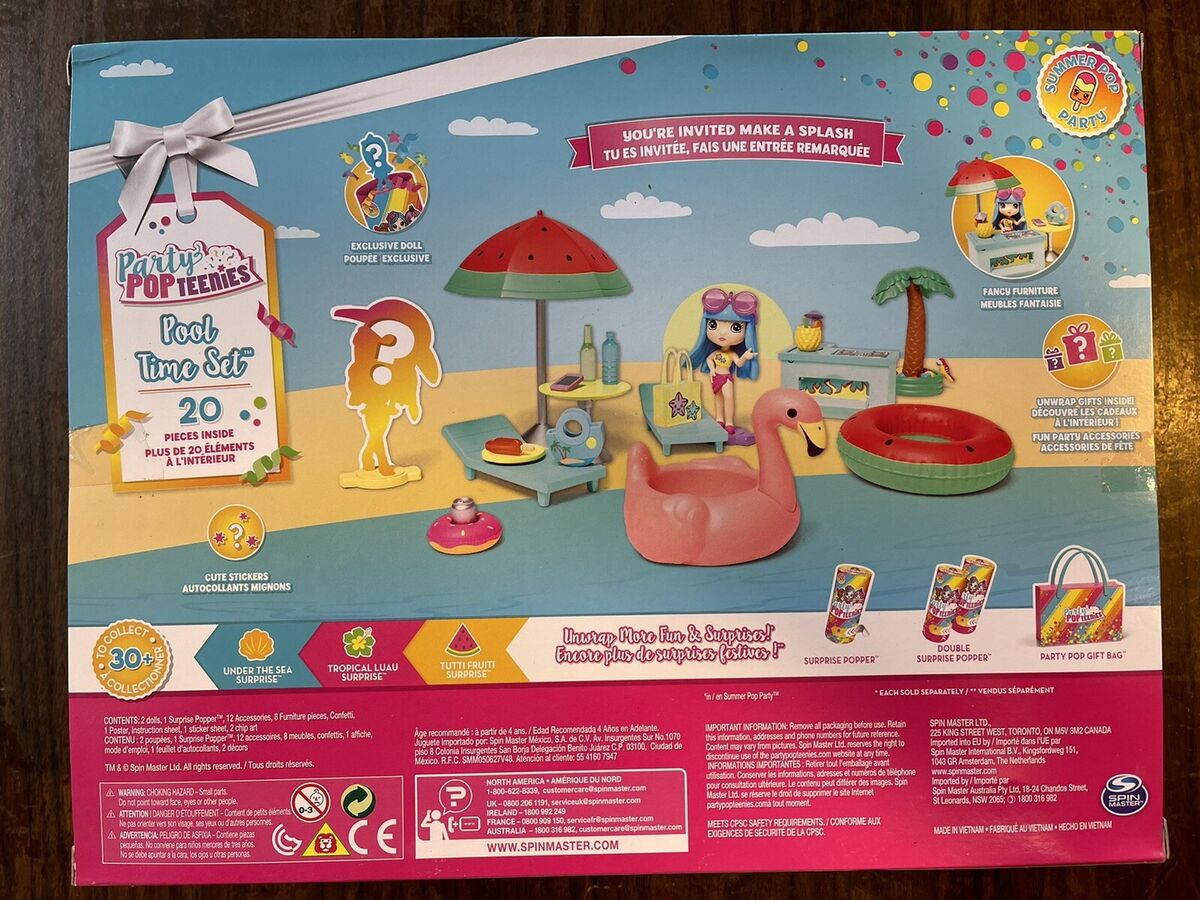The photograph showcases the colorful cover of the "Party Popteenies: Pool Time Set," a 20-piece toy for kids. The top two-thirds of the box features a vibrant cartoon beach scene with various playful elements. Central to this scene is a girl with blue hair and pink sunglasses, sitting next to a blue beach chair that has a green bag on it. Nearby, a yellow table with a watermelon-printed umbrella stands out, alongside a very light blue stovetop with a cartoon flame and a yellow pineapple with a small parasol. A brown cartoonish palm tree and assorted beach implements decorate the right side of the image.

The set includes fun poolside accessories such as a blue pool chair, a floating device with a watermelon print, a pink swan floatie with a hole for the doll, and a floating donut holding a white drink can. In the top left corner, a white background tag reads "Party Popteenies," followed by a blue-outlined text "Pool Time Set, TM" and the note "20 Pieces Inside." The top right corner features a confetti burst with a badge that says "Summer Pop Party," and a popsicle with a smiling face. Across the center top of the frame, a vivid pink band declares, "You're Invited to Make a Splash." The bottom section displays a pink background filled with white disclaimer text.